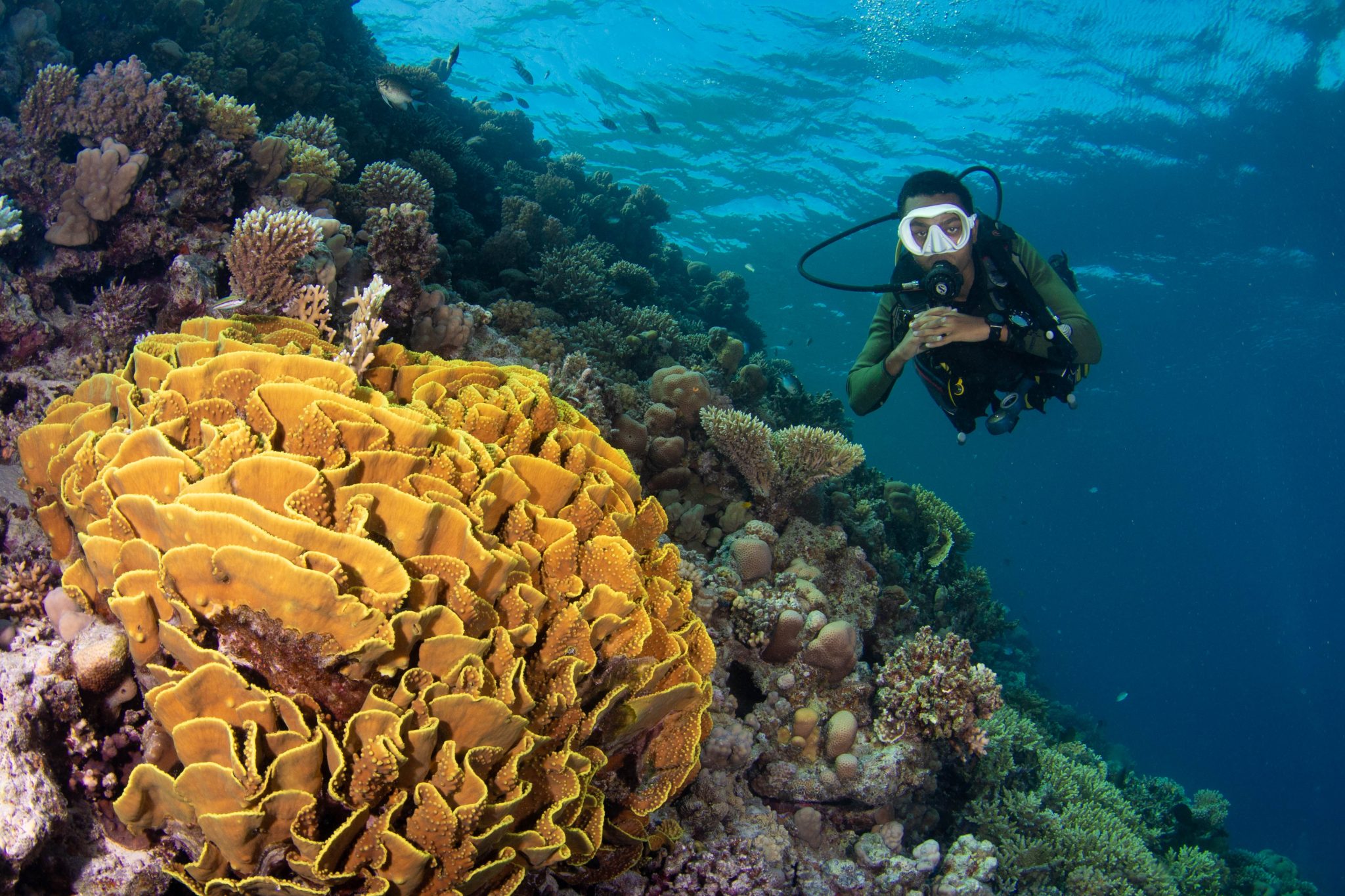In this underwater photograph, a snorkeler, who appears to be African-American, is swimming through a vibrant marine landscape. Wearing a green diving suit with a black breathing apparatus and white goggles, he navigates with his hands clasped in front of him. His black hair contrasts with the vibrant blue water that surrounds him, fading from light to dark blue as it deepens. 

The right side of the image captures his motion in the clear, reflective water. His scuba gear includes a watch on his wrist, and the regulator from his mouth connects to a tank on his back, facilitating his breathing. 

On the left, a diverse coral reef thrives with green, brown, and earthy tones. The reef creates a cliff-like structure sloping downward from the upper left to the lower right, with sections of the coral shifting from dark green to a more pinkish hue. A prominent, bright yellow piece of ribbony coral stands out in the lower left, resembling a large curly mushroom or cabbage. Amongst the coral, various fish swim near the lush underwater plants. The snorkeler appears to be swimming towards this rich, colorful ecosystem, highlighting the stunning biodiversity of the underwater scene.